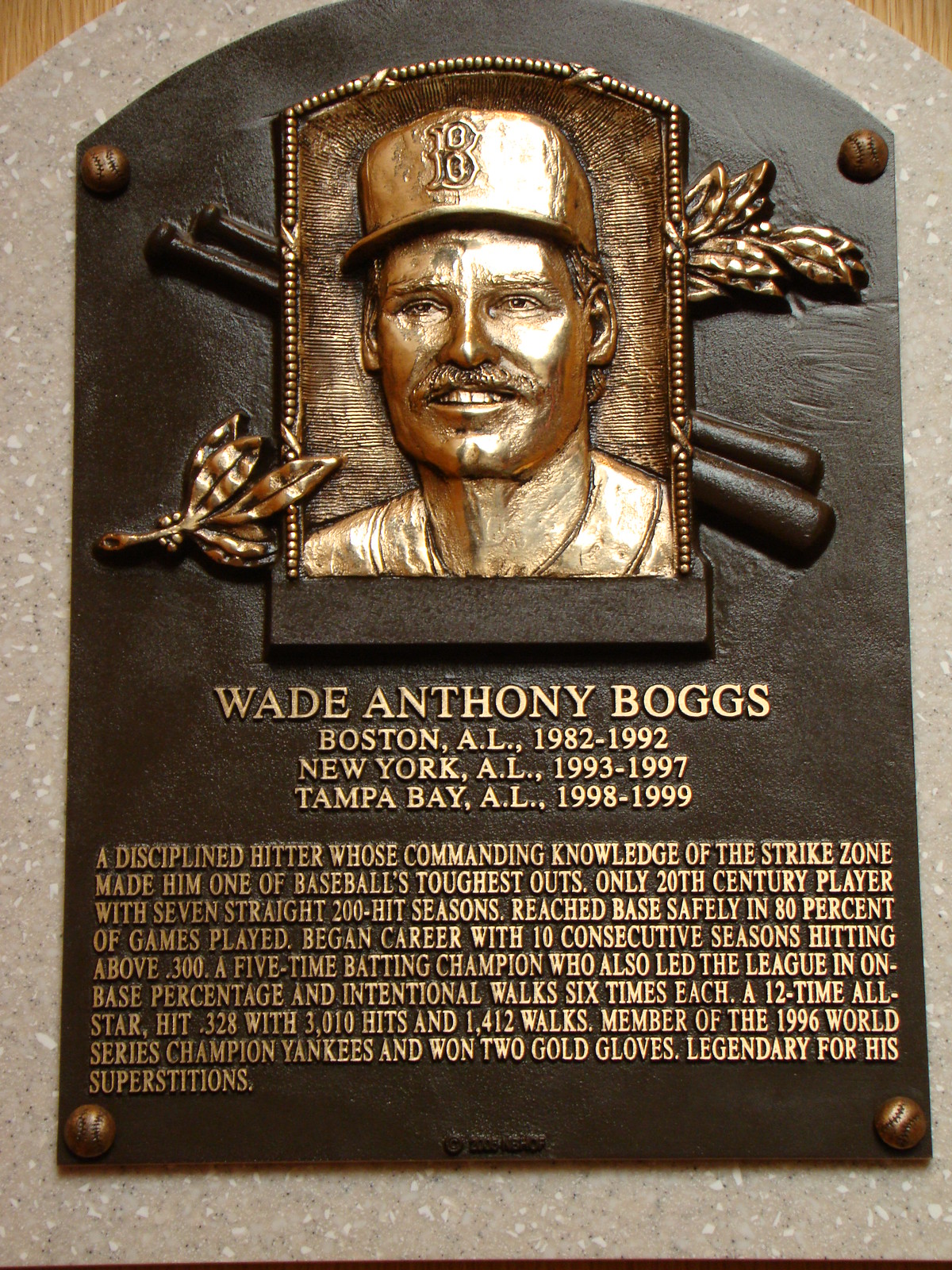This image depicts a bronze memorial plaque honoring baseball player Wade Anthony Boggs, designed in the shape of a headstone with a rounded top. The back of the plaque features a gray rock surface, to which a very dark brown plate is affixed with dark brown rivets resembling small baseballs. At the top center of the plaque is a detailed copper sketch of Wade Boggs's face, adorned with a mustache, slightly open mouth displaying his top row of teeth, and a baseball cap bearing the letter "B." His likeness is framed by flowers in the upper right and bottom left corners, as well as crossed baseball bats.

Below the portrait, his full name, Wade Anthony Boggs, is inscribed. The plaque documents his Major League Baseball career, specifying his tenure with different teams: Boston (1982-1992), New York (AL) (1993-1997), and Tampa Bay (AL) (1998-1999).

A long paragraph below this information highlights his exceptional career achievements. It reads: "A disciplined hitter whose commanding knowledge of the strike zone made him one of baseball's toughest outs. The only 20th-century player with seven straight 200-hit seasons, he reached base safely in 80% of games played. Began career with 10 consecutive seasons hitting above .300. A five-time batting champion who also led the league in on-base percentage and intentional walks six times each. A 12-time All-Star, he hit .328 with 3,010 hits and 1,412 walks. Member of the 1996 World Series champion Yankees and won two Gold Gloves. Legendary for his superstitions." All text on the plaque is in a dark copper color, providing a rich contrast against the dark brown background.